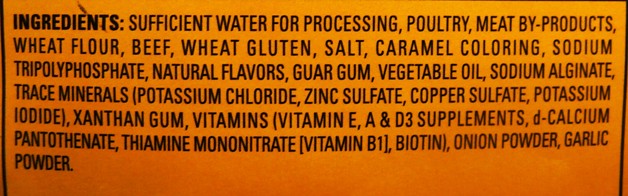The image depicts the ingredient list on an orange food product label. The top left corner prominently displays the word "INGREDIENTS" in bold black letters. The ingredients are listed in black capital letters and include sufficient water for processing, poultry, meat byproducts, wheat flour, beef, wheat gluten, salt, caramel coloring, sodium, tripolyphosphate, natural flavors, guar gum, vegetable oil, sodium alginate, various trace minerals, and different vitamins including vitamin E, A, D3 supplements, calcium pantothenate, thiamine mononitrate (vitamin B1), and biotin. Additionally, onion powder and garlic powder are also mentioned.